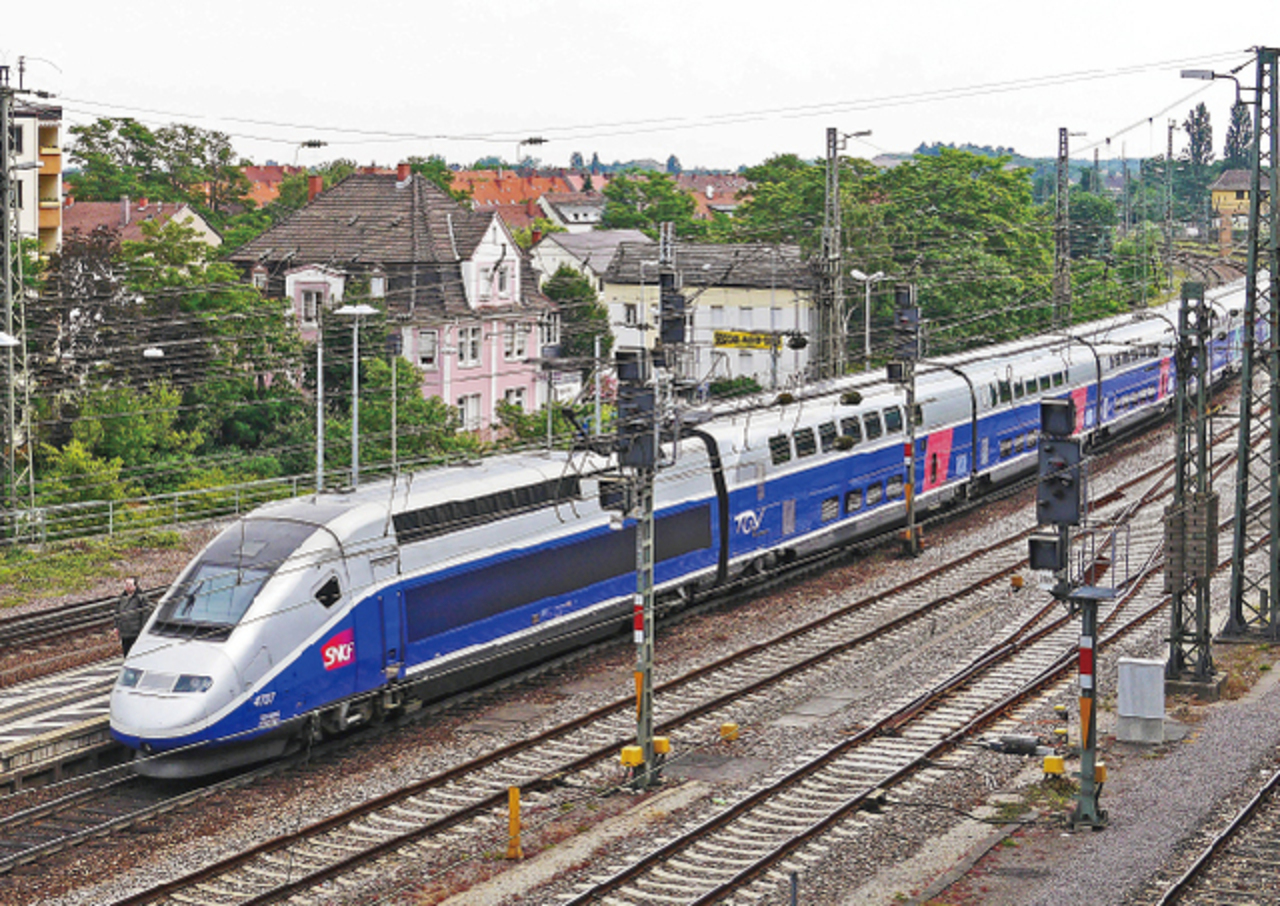In this detailed image taken from an elevated viewpoint, we see a long, two-story passenger train cruising through the scene, spanning nearly the entire photo. The train, distinguished by its dark blue lower base and silver upper section, features a large reflective windshield and prominent headlights at its front, which starts on the left-hand side of the image. The train runs on dark brown tracks with white horizontal pieces, alongside multiple sets of additional tracks visible at the bottom of the image. Surrounding the train are various infrastructural elements, including black poles and metal towers with light signals that are currently turned off.

To the left of the train, there are numerous houses painted in shades of pink, yellow, and white, many of which are multi-storied and topped with grey or orange roofs. Further to the right and in the background, more houses and rooftops can be seen amidst a mix of green trees on both sides of the track. The sky above is a pale white, suggesting an overcast day, with black power lines running through the upper portion of the scene. This combination of the train, houses, trees, and sky creates a dynamic and intricate composition.